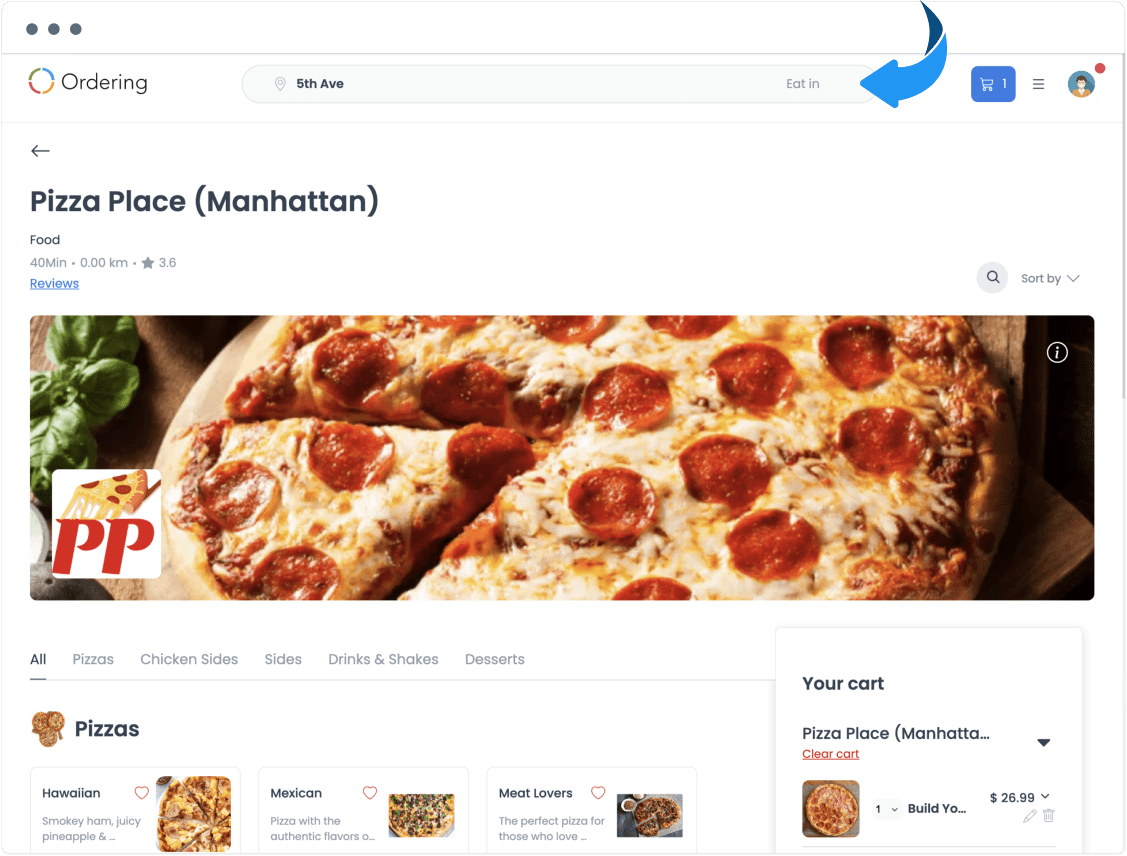Screenshot of a food ordering app showcasing a detailed mid-order for a pizza from "Pizza Place Manhattan." The interface, which appears on either a mobile device or a computer, features a prominent search bar at the top with the text "Eden" indicating the search function. The search bar displays "5th Avenue," suggesting the delivery location. A notification badge is present next to the profile picture, and there is one item noted in the shopping basket, indicating that the user has already started their order.

Centered on the screen is an appetizing image of a pepperoni pizza with one slice being lifted by a spatula, emphasizing its cheesy, greasy goodness. Above the image, in large black font, is the text "Pizza Place Manhattan." Beneath it are details about the restaurant: "Food, 40 minutes, 0 kilometers," and a 3.6-star rating with reviews available via a blue hyperlink.

Below the main image, various combo pizzas are listed, including Hawaiian, Mexican, and Meat Lovers. The user’s cart already contains one pepperoni pizza, possibly half cheese and half pepperoni, with an option to build your own pizza for $26.99.